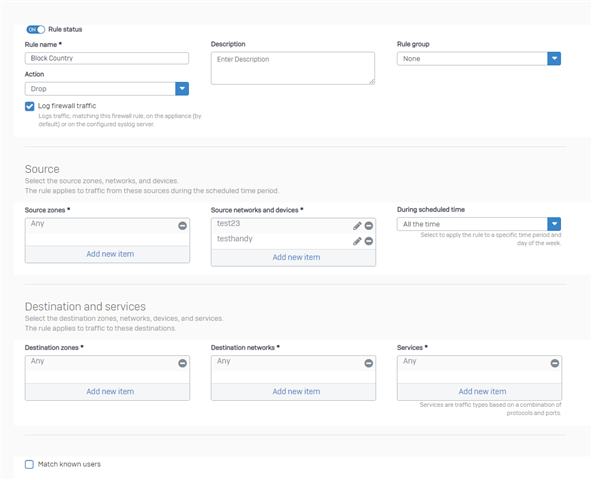### Detailed Caption for Firewall Rule Interface

The image depicts a detailed user interface for configuring firewall rules. 

- **Top Left Section:**
  - A toggle switch labeled **"Rule Status"** is turned on, indicated by its blue color.
  - Below it, a text field labeled **"Rule Name"** contains the value **"block country."**
  - Further down, the label **"Action"** is followed by the value **"drop"**, accompanied by a drop-down menu.

- **Checkbox and Logging Options:**
  - A checked box labeled **"Log Firewall Traffic"** is present. 
  - A description next to it reads: **"Log traffic matching this firewall rule on the appliance by default or on the configured log server."**

- **Right Section:**
  - A text field labeled **"Description"** prompts the user to **"Enter description"** in the data field.
  - Directly to its right, another label **"Rule Group"** shows **"None"** and includes a drop-down menu for selection.

- **Horizontal Divider:**
  - A horizontal line separates the upper and lower sections of the interface.

- **Source Configuration:**
  - The **"Source"** label indicates the settings for the zone, network, and devices the rule applies to during the scheduled time period.
  - The **"Source Zones"** field displays the value **"any"** with an option to **"Add New"**.
  - Below it, under **"Source Networks and Devices"**, two specific items are listed:
    - **"Test 23"**, next to which is a pencil icon inside a circle with a diagonal line.
    - **"Test Handy"**, similarly accompanied by a pencil icon inside a circle with a diagonal line.
  - At the bottom of this section is an option in blue: **"Add New Item."**